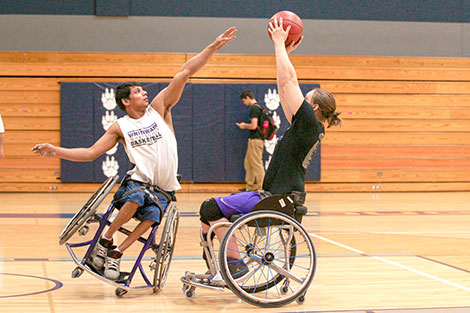The photograph captures an intense moment of a wheelchair basketball game being played on an indoor court. In the foreground, two players are in action. The player on the left, with short black hair, is wearing a white tank top, blue shorts, and black and white shoes. His purple wheelchair has silver wheels and a silver bar across the front. He is reaching high to his left, attempting to grab the basketball. On the right, his opponent, with brown hair tied back in a ponytail, is wearing a short sleeve black shirt, purple shorts, and gray shoes. He holds the basketball high over his head, trying to keep it away from the other player, while seated in his silver wheelchair.

The background features a young man who is not participating in the game. He has short black hair and is dressed in a black short sleeve shirt, khaki pants, and black shoes. He carries a black and red backpack and is focused on his cell phone. Behind him, there are wooden bleachers and a blue mat attached to the wall with white handprints. The setting is an auditorium with shiny light brown hardwood floors and brown wood walls. The upper part of the walls is gray and dark gray, and there is a dark gray banner with white paw prints on either side.